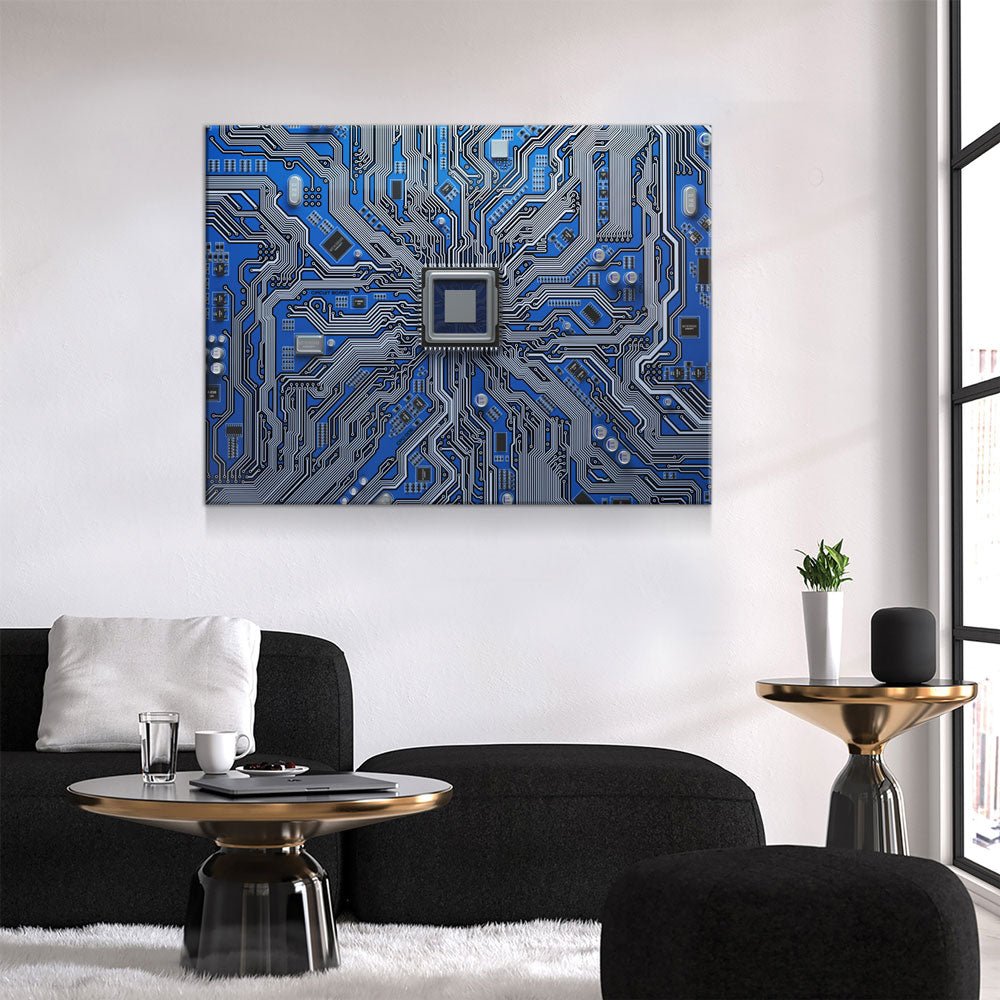This image showcases a modern, stylish living room with a striking focal point. Dominating the white wall is an elaborate 3D art piece, or possibly a highly detailed illustration, of a circuit board with a royal blue and gray color scheme. The design includes intricate circuits and a central square that almost looks like it could open up. Below the artwork, a sleek black sofa adorned with a single white throw pillow sits against a plush, shaggy white carpet. 

In the room's center is a low, glossy coffee table with a golden top and black base, holding a glass of water, a white coffee mug, and a slim laptop. A taller, matching side table stands between the sofa and a large floor-to-ceiling window on the right, featuring a white vase with green plants and what might be a smart speaker. Completing the furnishings are two black ottomans, adding to the minimalist yet chic ambiance of the room. The entire setup exudes a sense of luxury and modernity, enhanced by the bright lighting and expansive window.